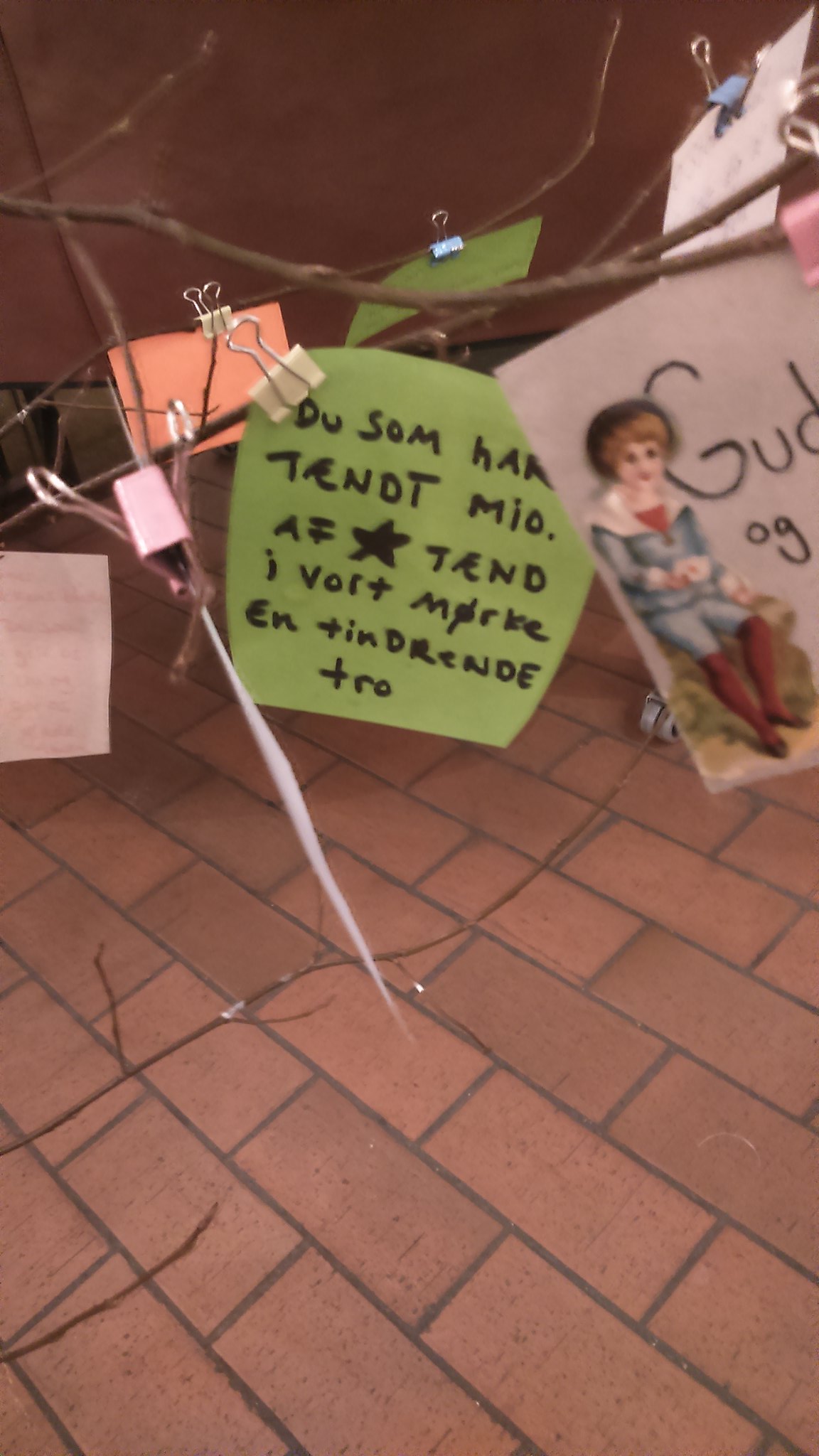The image depicts a chaotic scene with various elements attached to thin tree branches. These branches, possibly part of a small shrub, are placed in front of either a red brick concrete wall or a new and polished concrete floor with gray grout lines. Among the items clipped to the branches with blue, white, and pink paper binding clips are several colorful pieces of paper and sticky notes with handwritten texts. There is a prominent green sticky note with black writing that includes a star in the center and text resembling "Doosam, T-E-N-D-T-M-I-O," suggesting it could be in a different language, possibly Danish. Additionally, there is a note showing a background illustration of a seated figure, possibly a girl or a boy, along with the letters "G-U-D." In the foreground, another graphic of an illustrated Danish boy is partially visible. The overall impression is of an intricate, possibly outdoor display.